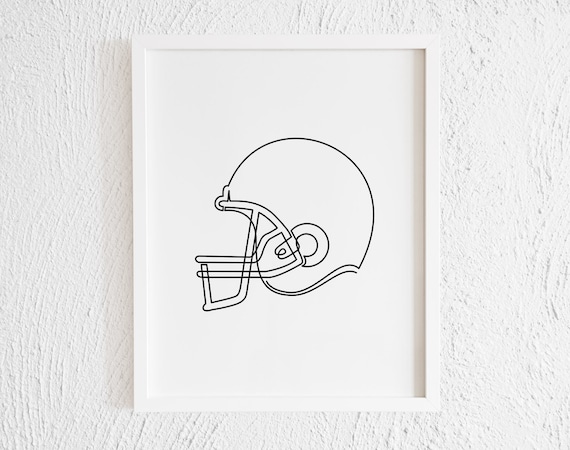The image showcases a framed, minimalistic line drawing of an old-school American football helmet, rendered in black outlines on white paper. The left side profile of the helmet is drawn with simple, elegant lines, including a face mask and ear hole. This sketch, which appears to use no more than ten lines, occupies about half of the paper, leaving the rest as negative space. The frame is a plain white wooden one, potentially sourced from a home decor store like Ikea. It's mounted on a textured white wall that adds subtle depth to the scene. Professional lighting ensures there are no distracting reflections, emphasizing the clean and simplistic aesthetic of the artwork.